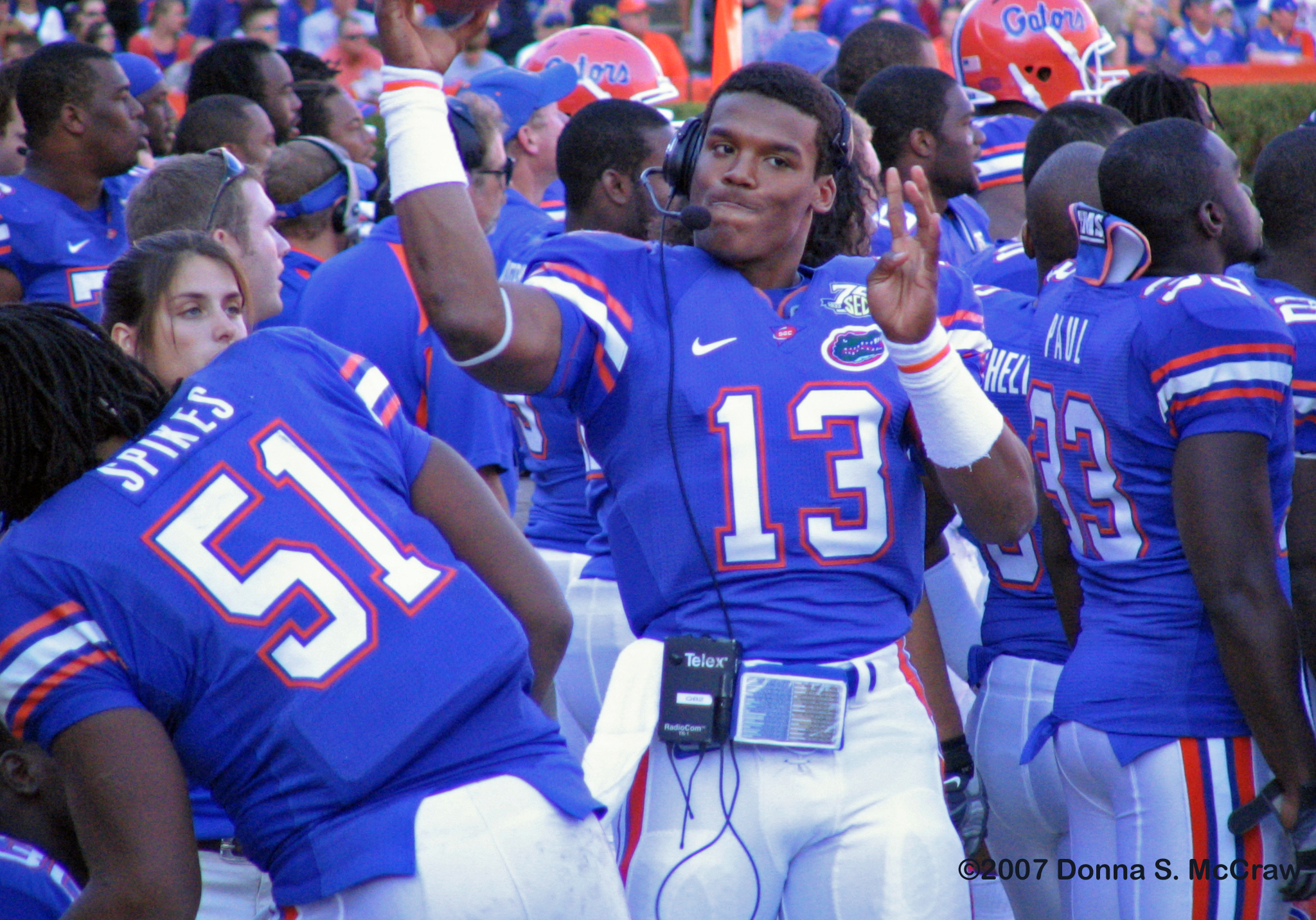The photograph depicts a dynamic scene from a football game, capturing a vibrant and intense moment. The focal point of the image is a football player, wearing a blue jersey with orange-red and white stripes, and white pants. He sports the number 13, and his last name is partially obscured but he's equipped with a headset—a common sight for those communicating with other play callers on the field. His right hand is raised in a gesture commonly associated with throwing a football, and his expression shows bemused concentration. Flanking him, to the left, is a teammate wearing a jersey numbered 51 with the last name "Spikes," and to the right, another player in jersey number 33, looking away.

Surrounding the central player are about 20 to 30 people, comprising teammates and coaches, positioned toward the foreground. All are intently focused in a specific direction, indicative of an ongoing game. The players are clad in matching blue jerseys with white pants, complete with white numbers bordered by the prominent orange-red and blue stripes. The background reveals an expansive crowd seated in stadium stands, contributing to the palpable atmosphere of the game. Amid the background, a green hedge is noticeable at the upper top right of the image. In the bottom right corner, the photograph is labeled with the copyright marking, "2007 Donna S. McCraw."